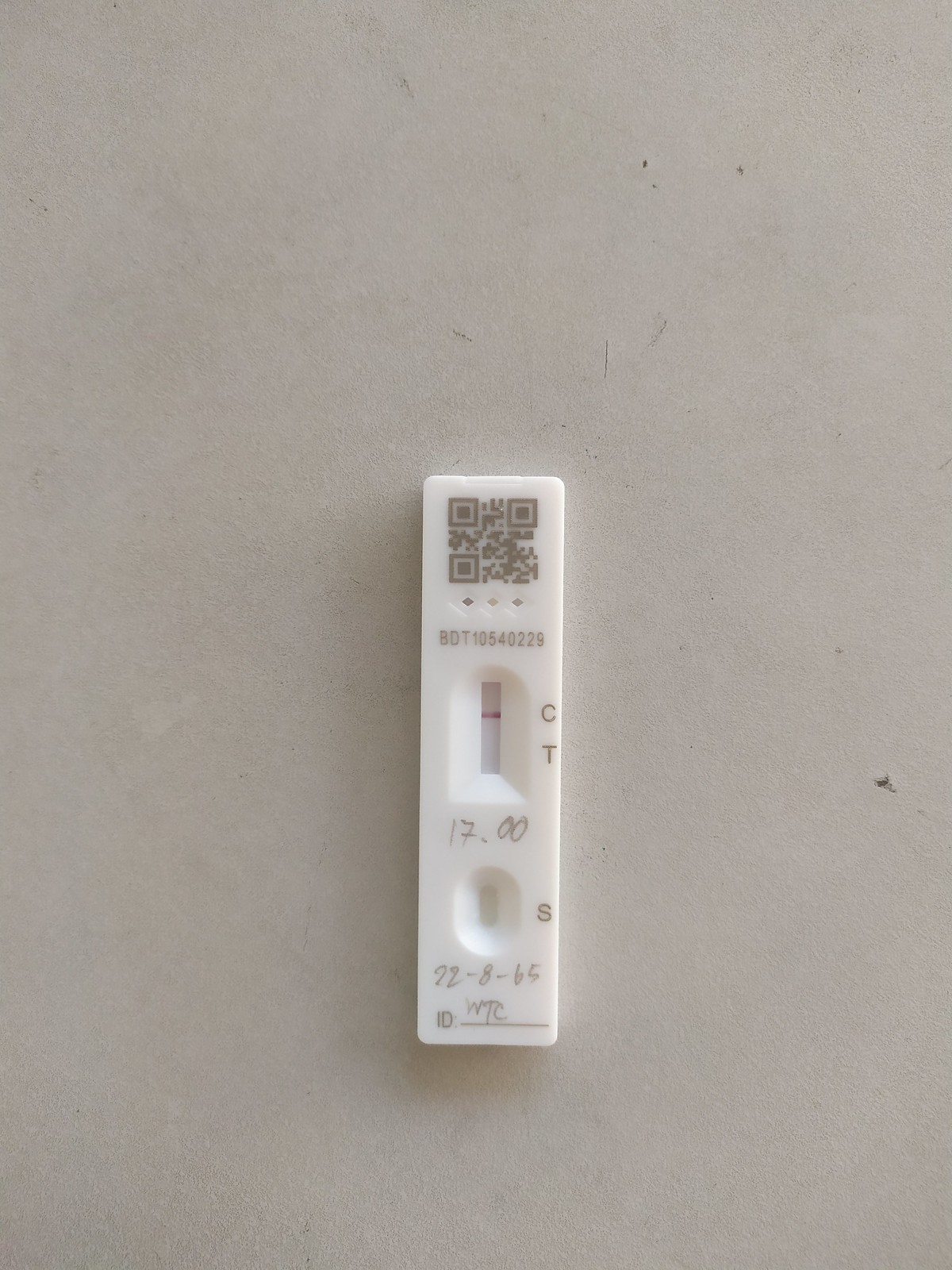The image depicts a vertically positioned, rectangular piece of plastic, likely a diagnostic testing device, possibly for urine analysis. The design bears some resemblance to common pregnancy tests but differs in several aspects. 

At the top, a QR code is visible, accompanied by some handwritten text. The primary section of the device features a small window displaying a red line, indicating a test result, labeled with the letter 'C'. Below this, the letter 'T' appears with no accompanying line. Further down is another window marked with 'S', which also lacks any visible line.

Handwritten annotations include the number '17.00' beneath the first section with the red line, and '72-8-65' below the section labeled 'S'. Additionally, there is a space labeled 'ID' and an illegible signature. The testing device rests on what appears to be a gray table.